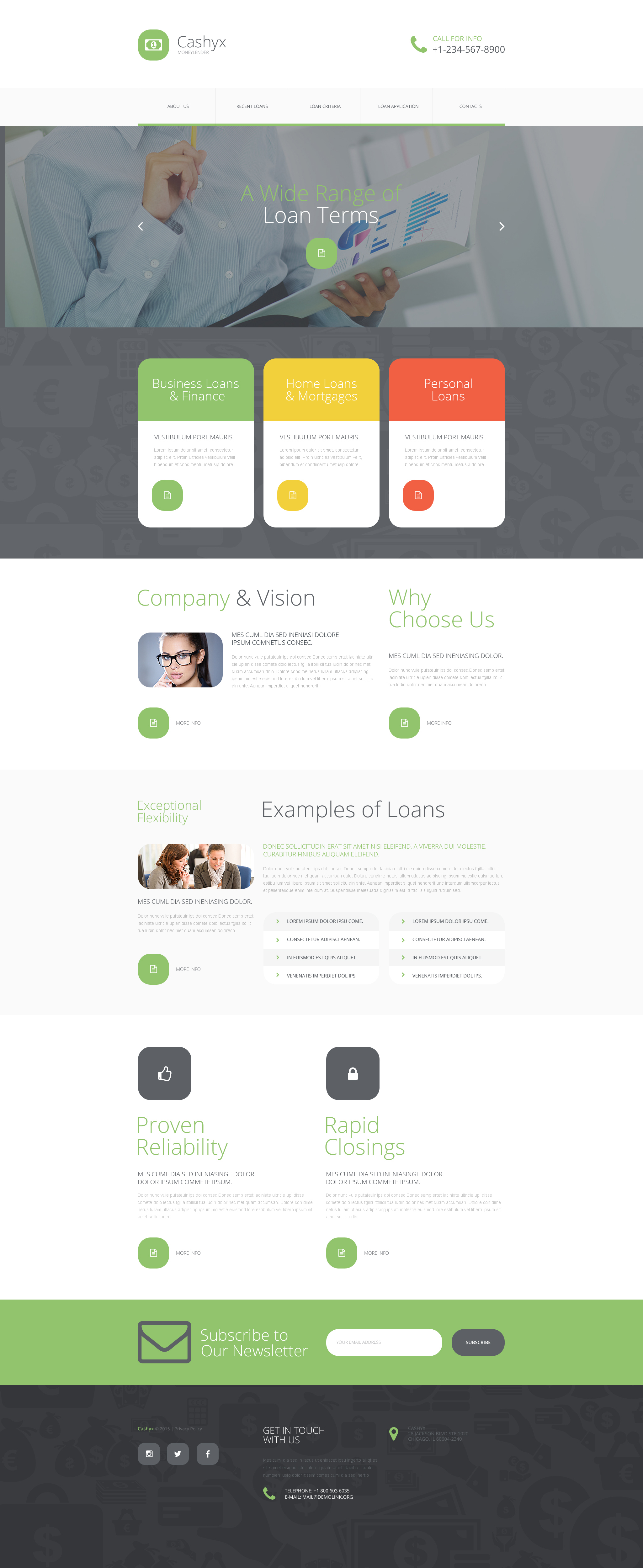This image is a screenshot of a webpage featuring various elements arranged vertically from top to bottom. At the top is a white banner that includes a small square red icon with an icon resembling a white dollar sign, though the details are hard to discern due to its size. To the right of this icon, the text "CASHYX" is displayed in black font. Further to the right, there is an old-fashioned telephone handset icon with the accompanying text "Call Us" and the phone number "1-224-567-4800."

Below the white banner, a gray rectangle contains five menu items written in black font, but they are too small to read clearly. Beneath this is a graphic of a woman dressed in a button-up collared blue shirt. She is holding an open white folder in her right hand, which contains white paper featuring blue text. Superimposed above this image is the text "A wide range of loan terms." Additionally, a small yellow circle with a barely visible white icon is present within the graphic.